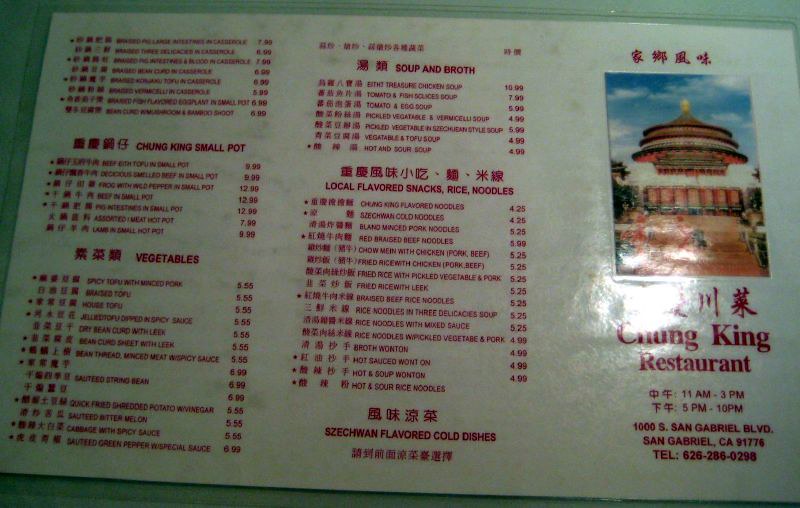This is a photograph of a laminated, rectangular menu from Chung King Restaurant, located in San Gabriel, California. The menu has a white background with red lettering and features the restaurant's name, location, address, and telephone number on the right side. An image of an Asian pagoda with a brown roof and a golden top against a blue sky is prominently displayed, with Chinese characters above it.

The menu is organized into several sections, including Small Pots, Vegetables, Soup and Broth, Local Flavored Snacks, Rice Noodles, and Sichuan-Flavored Cold Dishes. Each section lists various dishes in both Chinese and English, accompanied by their respective prices on the right. The photo appears to have been taken on a white tabletop, providing a clean and clear view of the menu's details.